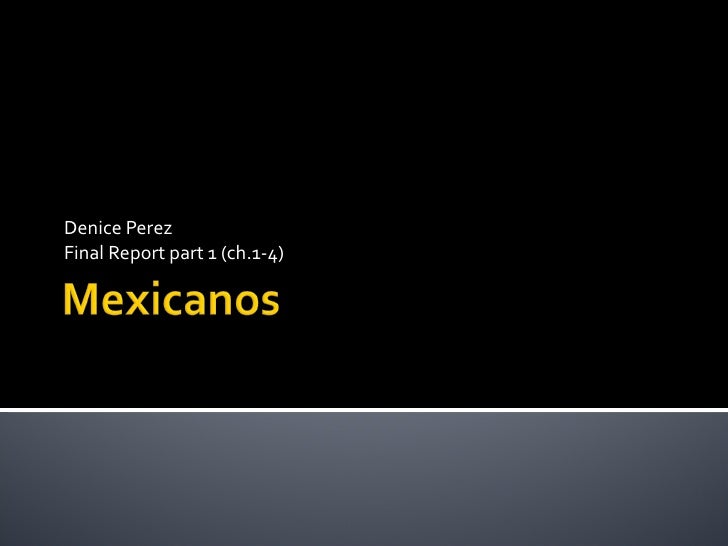The image depicts a basic slide, likely from a PowerPoint presentation, set against a vast black background. Dominated by minimalistic design, the slide features a gray gradient bar spanning the bottom, subtly lighter in the center and darker at the edges. In the bottom left corner of the frame, white text reads "Denise Perez, Final Report, Part 1, Chapter 1-4," while a bold yellow word, "Mexicanos," stands out beneath it. The setting suggests an academic context, with the layout emphasizing the sparse, empty black space around the text and bar, drawing attention to the key details presented.